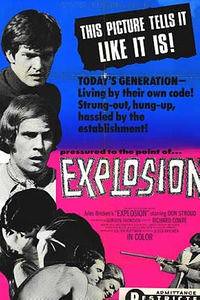This movie poster, reminiscent of an era gone by, dramatically captures the tumultuous spirit of its time. The top half of the poster is dominated by a stark blue background, with a bold black section in the top right corner proclaiming in white text, "This picture tells it like it is." Below, black text reads, "Today's generation living by their own code, strung out, hung up, hassled by the establishment." To the left, there are striking black-and-white images of various men, one with dark hair contorted in an expression of either anger or confusion, and another with slightly longer hair, enhancing the vintage feel. The bottom half transitions into a vivid hot pink backdrop with the compelling phrase "pressure to the point of explosion" in black text, culminating in the word "EXPLOSION" in bold white lettering. A dynamic collage of imagery overlays this section: a man and woman kissing, a scene of nudity, and a woman brandishing a gun in the lower right corner, hinting at a narrative of rebellion and unrest. Despite some text being too blurry to decipher, the overall impression is unmistakably that of a gripping, provocative movie poster.